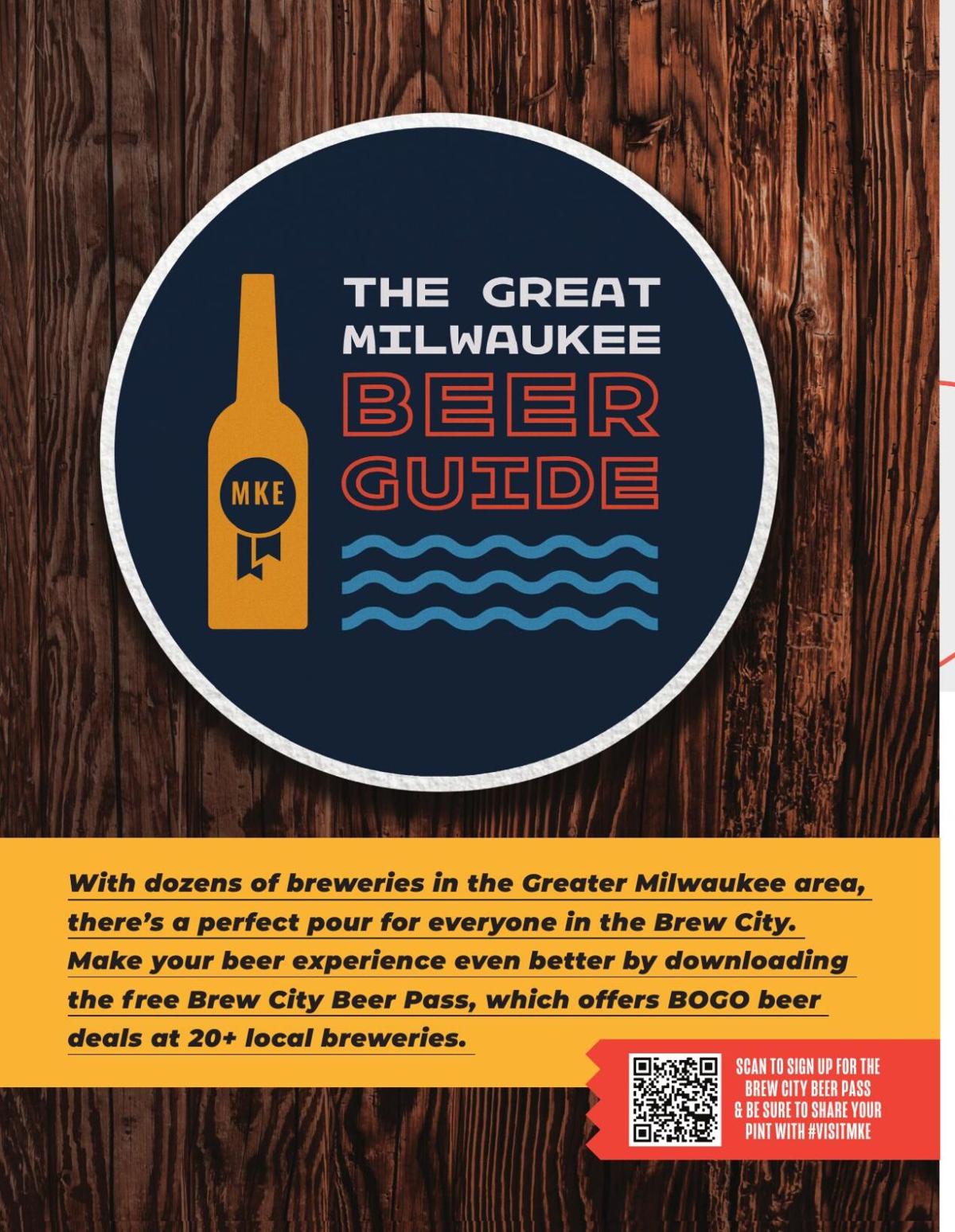This is a digital advertisement poster set against a dark wood-grain background with deeper textured accents. Dominating the top two-thirds of the image is a navy blue circle outlined in white, featuring the title "The Great Milwaukee Beer Guide." The phrase "The Great Milwaukee" is rendered in white text, while "Beer Guide" is showcased in a bold, orange, and dark blue font. Beneath the text are wavy blue lines, adding a playful touch to the design. To the left of the text, there's a gold-colored beer bottle, enhancing the theme. 

Continuing below, a yellow bar stretches across the poster, stating, "With dozens of breweries in the Greater Milwaukee area, there's a perfect pour for everyone in the Brew City." This is followed by an enticing call to action: "Make your beer experience even better by downloading the free Brew City Beer Pass, which offers buy one get one BOGO beer deals at 20 plus local breweries." Finally, in a small orange square at the bottom right is a QR code, accompanied by some illegible white text, allowing viewers to easily sign up for the Brew City Beer Pass.